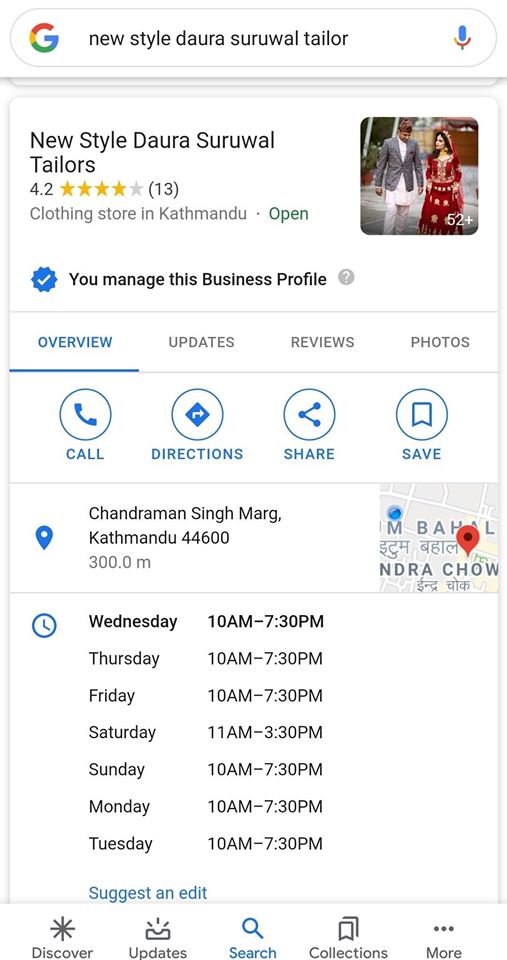The image shows a Google search result for "New Style Dori Saral Taylors," a clothing store located in Kathmandu, India. The Google Chrome interface is visible with an icon signifying Google on the left, characterized by its distinctive rainbow colors. To the right, there's a microphone icon indicating the voice search option.

Prominently displayed is the business profile of New Style Dori Saral Taylors, showing a review rating of 4.2 stars based on 13 reviews. The store is highlighted as open, indicated by a green status label. A series of images are shown, featuring individuals in various traditional attires: a woman in a decorative red dress, and a man in a long white shirt worn with a blazer. A total of 52 images are available to browse.

The page indicates that the user managing the business profile has access to manipulate the information, as indicated by a check mark. The profile's "Overview" section is currently visible, with accessible options such as call, directions, share, and save. The physical address of the store is shown as being 300 meters away, alongside a Google Maps panel pinpointing its location within Kathmandu.

The store's operational hours are listed, indicating it is open from 10 AM to 7:30 PM Monday through Tuesday, and from 11 AM to 3:30 PM on Saturdays. At the bottom of the screen, various options such as Discover, Updates, and Collections are available, with the current focus on the Search feature, indicated by a metal icon.